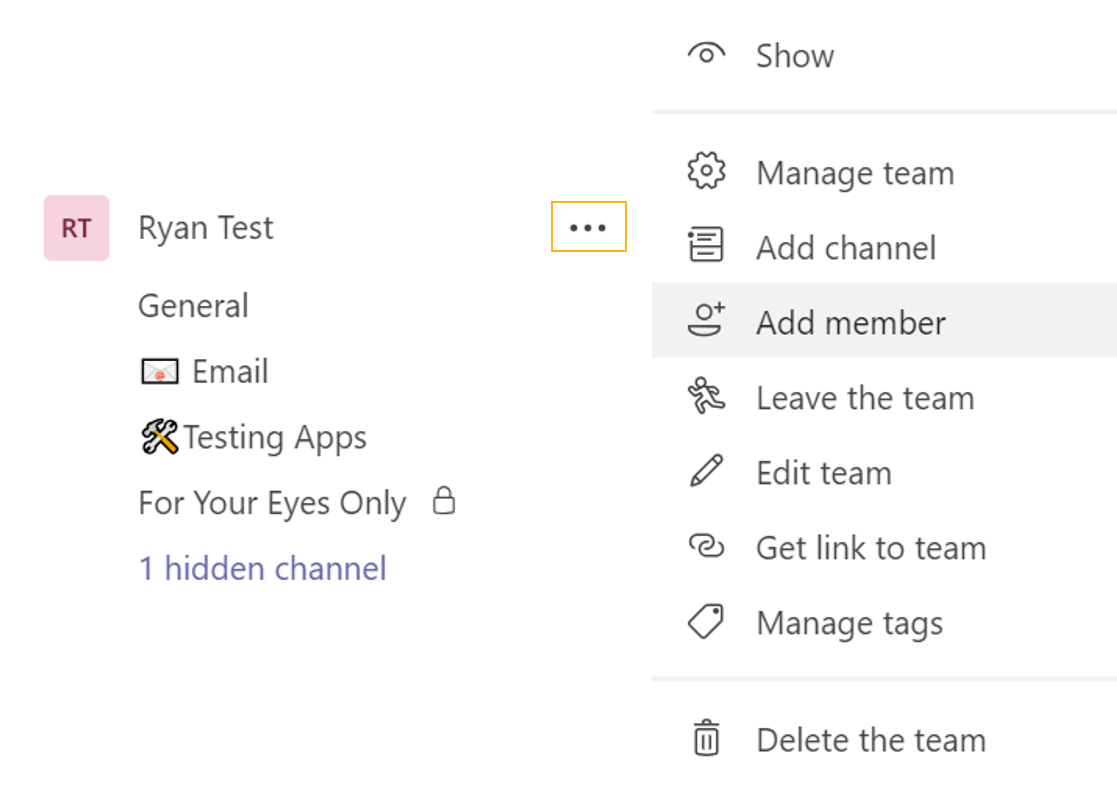The image shows a computer screen displaying a software interface. The main section in the center of the screen has a white background. On the left side, there is a vertical menu bar.

The most prominent feature on the page is a section labeled "RT," which is highlighted in red with a pink background, contrasting with the rest of the page's white background. To the right of "RT," there is a title labeled "Ryan test." Below "Ryan test," the text reads "general email testing apps." 

For the "email" category, there is a page icon. For the "testing app" category, there is a settings icon depicting a hammer and a wrench. Below these categories, the text reads "for your eyes only" accompanied by a lock icon, indicating restricted access. Further down, there is a note saying "one hidden channel," with this text colored in blue.

At the center of the page, there are three black dots surrounded by an orange outline square, presumably a menu or settings icon.

On the upper right side, the text "show" is displayed, with a drop-down menu listing several options, each with specific icons: 
1. "Manage team" with a gear icon.
2. "Channel" with a list icon.
3. "Member" with a plus sign icon.
4. "Leave the team" with a running character icon.
5. "Edit team" with a pencil icon.
6. "Get link to team" with a chain link icon.
7. "Manage text" with a tab icon.
8. "Delete the team" with a trash bin icon.

The layout is organized and each icon is clearly associated with its respective function, providing a detailed and navigable interface.